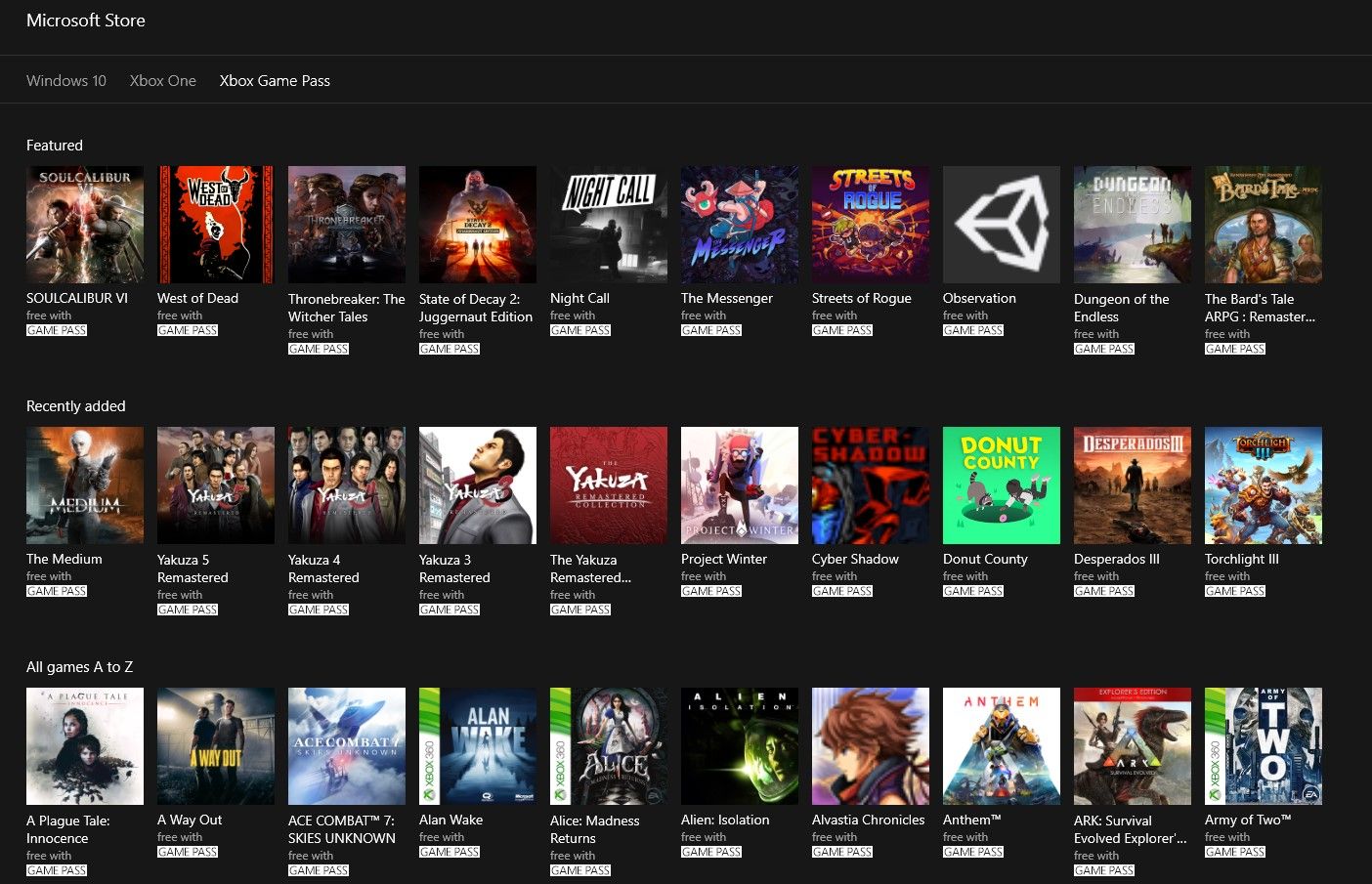The web page from the Microsoft Store showcases various games available for purchase, presented in colorful cover designs against a dark gray or black background. At the top of the screen, "Microsoft Store" is prominently displayed in white text. Below this, a menu bar offers three selections: Windows 10, Xbox One, and Xbox Game Pass, with Xbox Game Pass highlighted in a brighter white.

In the main section of the page, there are three rows of content. The top row, labeled "Featured" in white text, displays ten different games. The middle row, titled "Recently Added," features five new game releases. The bottom row is an "All Games A to Z" section, displaying additional games along with their cover art and titles. 

Under each game's title, a description states "free with," followed by "Game Pass" highlighted in a large, bold white text, emphasizing that these games are available at no additional cost for Xbox Game Pass subscribers.